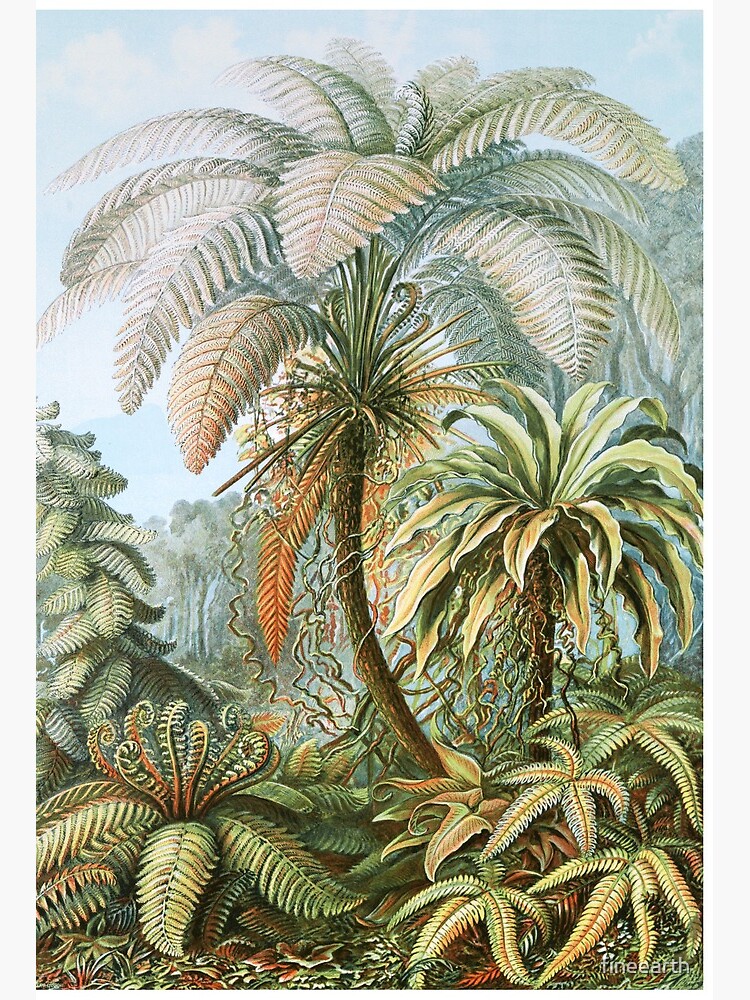This artwork, a fanciful and vibrant digital painting, captures a tropical scene with a prominent central palm tree. The tree, adorned with lush green and gold leaves, features a trunk draped with vines and hanging golden fronds. Adjacent to the main tree, a slightly smaller palm can be seen on the right. The ground below hosts various plants, some resembling starfish with similarly designed leaves, possibly early growths of larger flora. On the left side, a tall stack of smaller leaves adds to the dense vegetation. The background presents a clear blue sky, enhancing the tropical ambiance. Rich with colors including green, light blue, grey, red, orange, and white, the composition is artistic and imaginative. The bottom right corner contains the text "Vintage wall art," emphasizing its decorative and nostalgic charm. The whimsical nature of the scene, with hints of wilted yellow leaves among the green, suggests an artistic interpretation rather than a realistic portrayal, giving the piece a unique, wavy, and almost surreal quality.